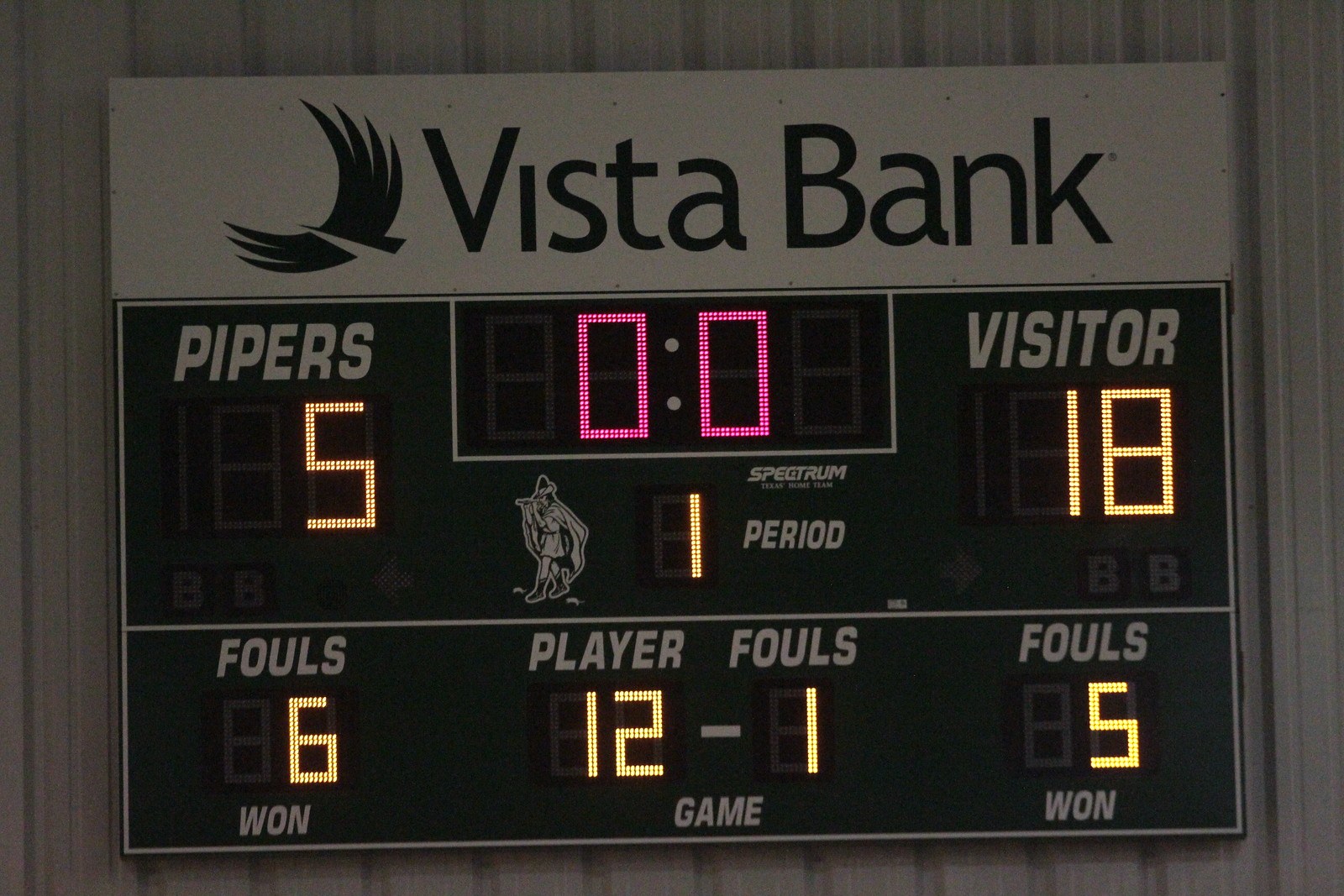The image is a close-up of a scoreboard, prominently displaying the text "Vista Bank" in green lettering with an abstract bird logo featuring spread wings. The background of the scoreboard is primarily white metal with a dark gray border. The scoring area has a green backdrop. On the left side, the scoreboard shows "Pipers" in bold white letters, with a lit-up score of 5 underneath. On the right side, "Visitor" is also in white letters, displaying a score of 18. In the center of the scoreboard, red-lit zeros indicate the time, while "Period 1" is written below this, featuring a small character image next to the number 1. The lower section of the scoreboard includes the word "Spectrum" beneath the zeros. At the bottom left, it indicates 6 fouls for Player 12 of the Pipers team, and to the right, it shows 5 team fouls for the Visitor team.